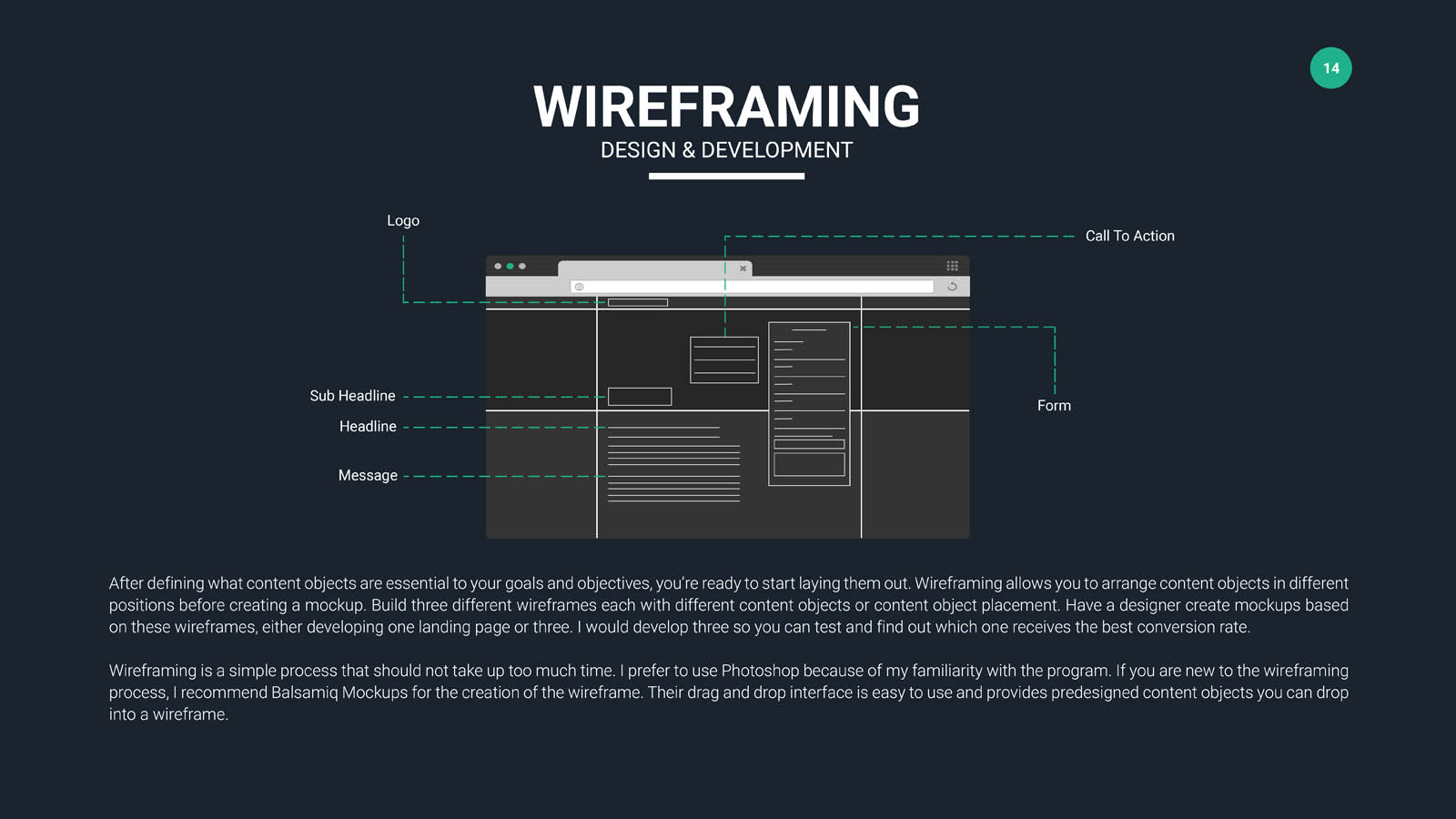The image, titled "Wireframing Design and Development," features a detailed schematic of a wireframing design process against a dark blue background. At the top, the title "Wireframing Design and Development" is displayed in white block text with various font sizes. A white line separates the title from the central rectangular wireframe diagram, which is composed of grey and white lines and boxes. 

In the top left of the wireframe diagram, there's a "logo," with a "subheadline" and "headline" positioned below it. At the lowest part on the left, a "message" is indicated. The right side of the diagram includes sections labeled "call to action" and "form." Teal dashed lines connect these labels to their respective components within the diagram.

In the upper right-hand corner of the entire layout, there is a teal circle with the number 14 written in white. Below the diagram, two paragraphs of text describe the wireframing process. Although the text is small and somewhat faint, it emphasizes the importance of arranging contact objects before creating a mock-up, and suggests creating multiple wireframes to test for the best conversion rate. The finer details also share personal preferences and recommendations for wireframing tools, such as Photoshop and BASEMIC mock-up, particularly noting the ease of use provided by BASEMIC's drag-and-drop interface.